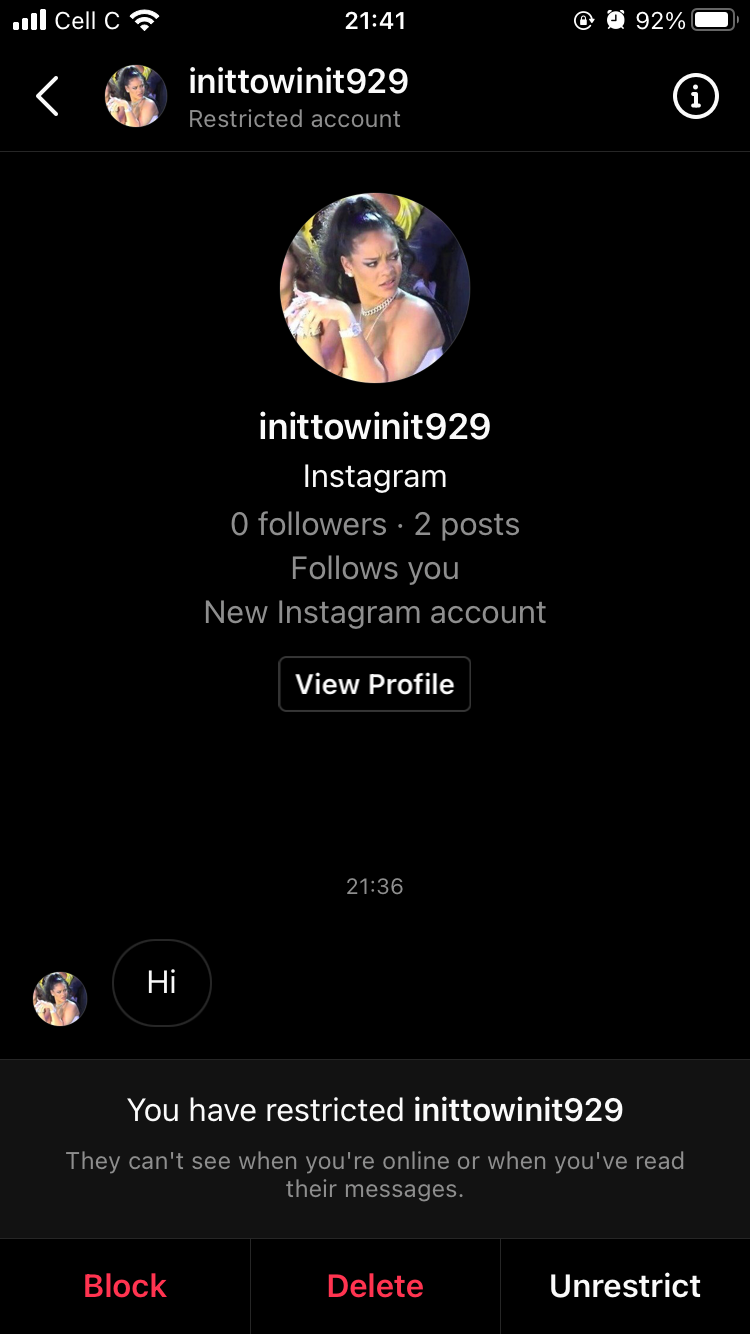"Screenshot of a mobile phone displaying the home screen with a detailed view of various notifications and icons. The status bar at the top shows full cell service bars, active Wi-Fi connectivity, the time as 21:41, and a 92% battery level. The phone has restricted notifications, indicated by a status message, 'In it to win it nine to nine,' suggesting limited communication features. 

On the screen, an Instagram-related notification mentions 'zero followers' and options like 'unrestrict,' 'view profile,' 'high block post,' and a 'follows you' message for a new Instagram account. There is also a white circle with an eye icon, multiple generic profile pictures, and text in white and gray letters against a black background, emphasizing an interaction with Instagram's privacy and notification settings. Everything is organized in a typical smartphone interface layout."